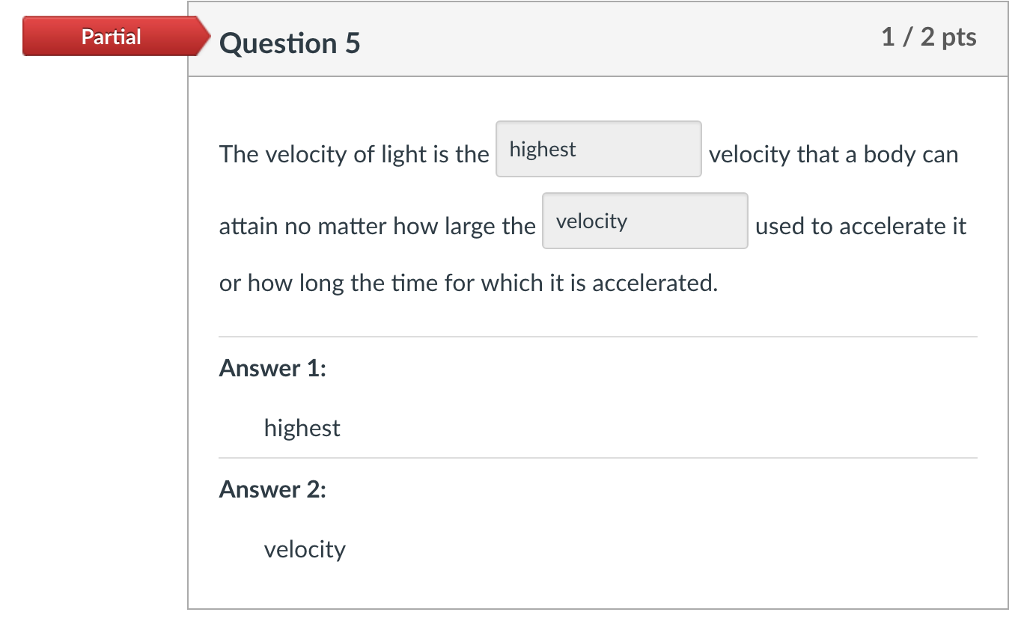The image is a partial screenshot of a question section from a website. In the top left corner, there is the word "partial," indicating that the image does not capture the entire page. The main feature of the image is a rectangular box with a pointy end on its right side, which directs attention to "Question 5," bolded, and also located near the top left corner of an overlapping square.

"Question 5" is displayed in a light gray banner. To the right of the banner, the notation "1/2 PTS" indicates that the question is worth 1 out of 2 points. Below this banner, the question text reads: "The velocity of light is the highest," with the word "highest" framed within a gray rectangle box, followed by, "velocity that a body can attain no matter how large the velocity or how long it is accelerated."

A horizontal line separates the question from the answer section. "Answer 1:" is bolded, followed by the response "highest." Another horizontal line separates this answer from "Answer 2:" which is also bolded. The response under this second answer is "velocity."